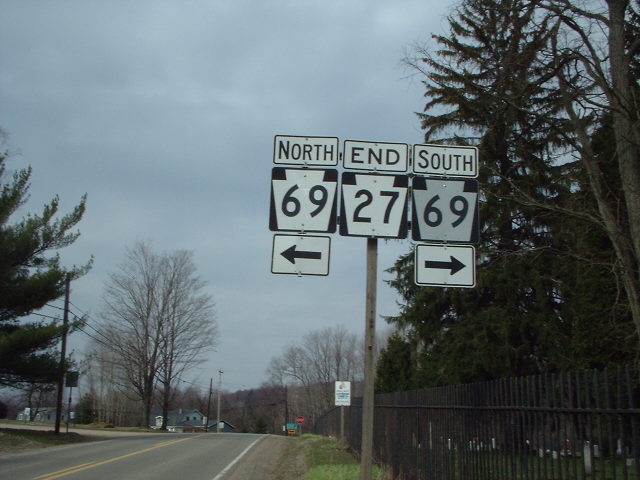The landscape-format color photograph depicts a side view of a two-lane road, clearly showing a prominent traffic sign pole with three distinct signs. The left-facing arrow indicates "North 69," the middle sign reads "End 27," and the right-facing arrow points to "South Route 69." Set against a backdrop of a semi-cloudy sky, the scene suggests a cold day, as the deciduous trees are bare while the coniferous ones retain their needles. A dark iron fence runs along the right side of the road, potentially enclosing a cemetery. Multiple signs, including a distant stop sign and possibly green and yellow signage, are also visible. Wooden houses or buildings are discernible in the background, and a mix of dead and evergreen trees lines the road and fence. The setting is further characterized by power lines running parallel to the road and the noticeable change in the surroundings beyond the fence, highlighting the separation between the road and the areas it navigates.